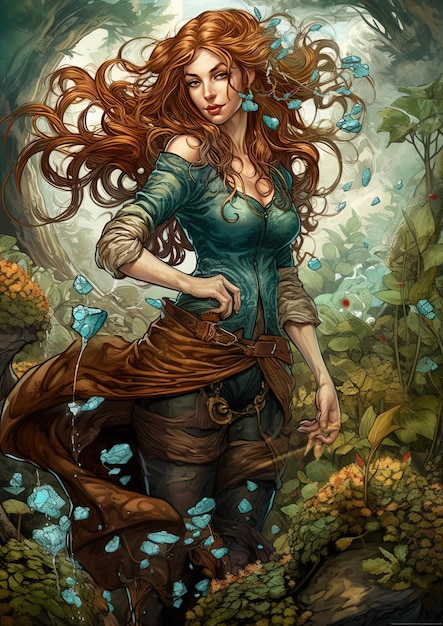A detailed, descriptive caption:

This ornate rectangular painting portrays a sensuous woman with voluminous, flowing orange-brown hair that reaches down to her waist, wavy and carried by a breeze. The backdrop is lush and almost waist-high green shrubbery, with scattered bright blue flowers and varying green leaves, creating a dense, forest-like atmosphere. At the center, we see the woman from her knees up, standing amidst the greenery that covers the very bottom of the scene. Her head, tilted slightly to her right, reveals a serene, closed-lip expression. She is dressed in a tight-fitting, teal blue top that exposes her cleavage and her right shoulder, with sleeves that extend barely past her elbows. Her right arm is bent, placing her hand on her hip, while her left arm, also bent, drapes down below her waist. She wears dark charcoal-grey pants, complemented by a long brown cloth tied around her waist, fluttering in the wind and mirroring the movement of her hair. The composition includes a circular light behind her, framed by two tree trunks like an otherworldly aura, enhancing the enchanting and almost magical presence she exudes.